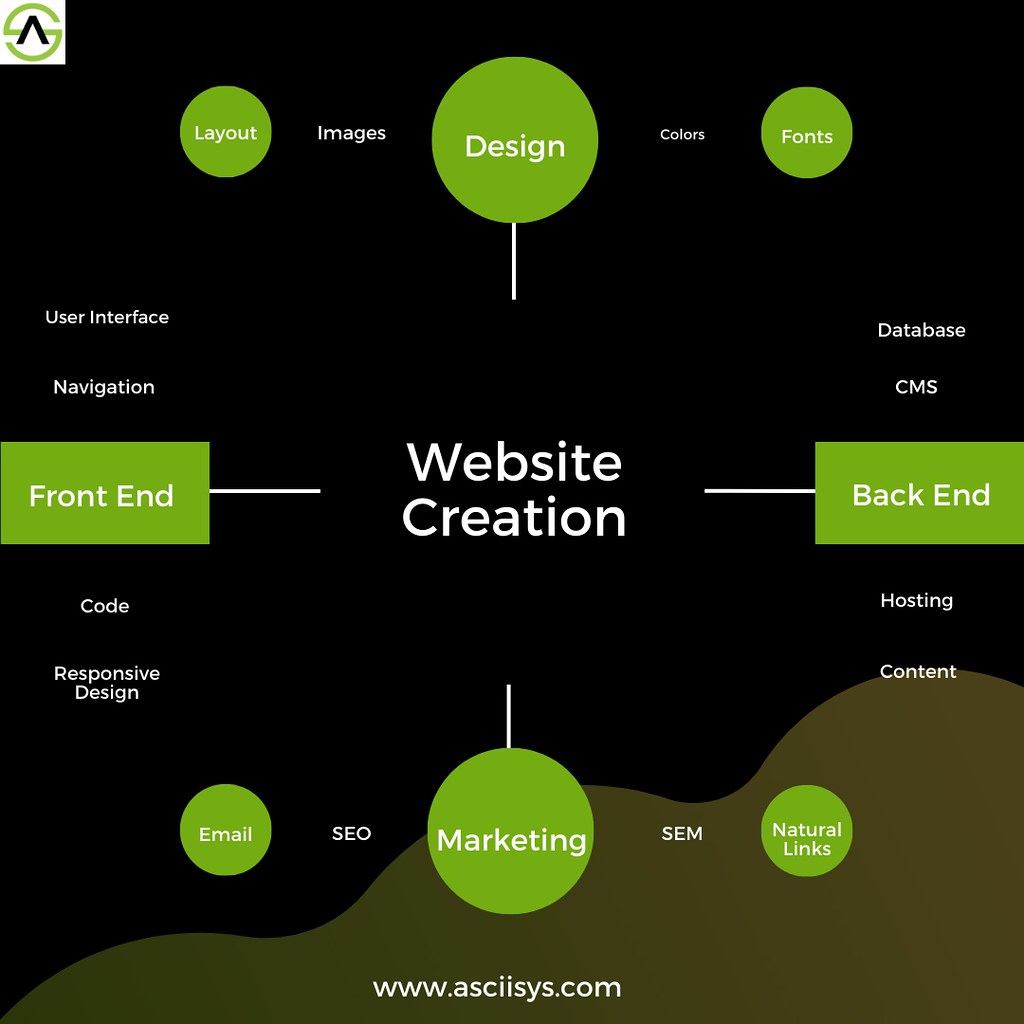The image depicts a detailed website creation diagram set against a black backdrop with olive green hills on the lower right corner. Central to the diagram is a significant green circle labeled "website creation." At the top, three circles are present: a small one labeled "layout," a larger circle saying "design," and another small one labeled "fonts." On the bottom, moving left to right, are small green circles reading "email" and "natural links," and a large central circle stating "marketing." 

On the left side, a green rectangle labeled "front end" sits midway, with vertical text to its left listing "user interface," "navigation," "code," and "responsive design." On the black background, other elements include "images," "colors," "SEO," and "SEM." 

On the right side, a similar green rectangle reads "back end," flanked by vertical text listing "database," "CMS," "hosting," and "content." The design overall emphasizes the structure and components essential for creating a website, with each element clearly marked and connected by white lines. At the bottom of the image, the website "www.asciisys.com" is displayed.